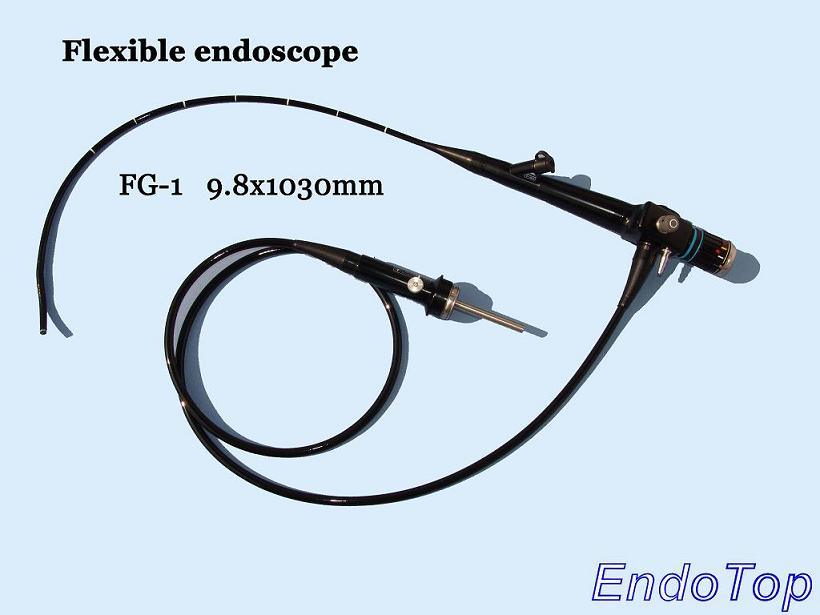This is a detailed photograph of a medical device, specifically a flexible endoscope. The image prominently features the endoscope coiled on a light baby blue surface. The endoscope, primarily black, resembles a whip in design with two distinct wires extending from it. One wire curves upwards from the handle, while the other wire loops midway between the handle and the distal end. The device tapers from a handheld section, which likely contains dials for maneuvering, into a thinner, sleek, flexible portion ending with a precision tip. The text in the image includes "Flexible Endoscope" in the top left corner and the specification "FG-1 9.8 x 1030 mm" inscribed along the endoscope. Additionally, the bottom right corner features the word "Endo Top" in dark blue outlined lettering, which could be the brand name. All textual elements are in black except "Endo Top."